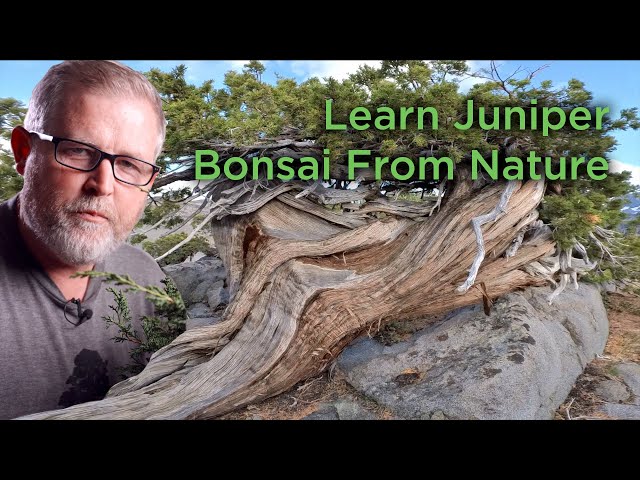This color photograph, likely a YouTube thumbnail or magazine cover, features an outdoor scene on a clear day. The text "Learn Juniper Bonsai from Nature" is prominently written in green at the top right. The photo captures an older gentleman, around 60 years old, standing to the left. He has grayish-white hair and a full beard and mustache of the same color. He wears black glasses and a gray t-shirt with a microphone attached. The man appears to be squinting and has a slight frown as he looks at a large juniper bonsai tree laying on a rock. Multiple bonsai trees and scattered stones and driftwood, possibly juniper, are visible in the background, all set under a clear blue sky. The scene suggests that the man is likely a YouTuber or presenter explaining how to grow juniper bonsai trees from nature.